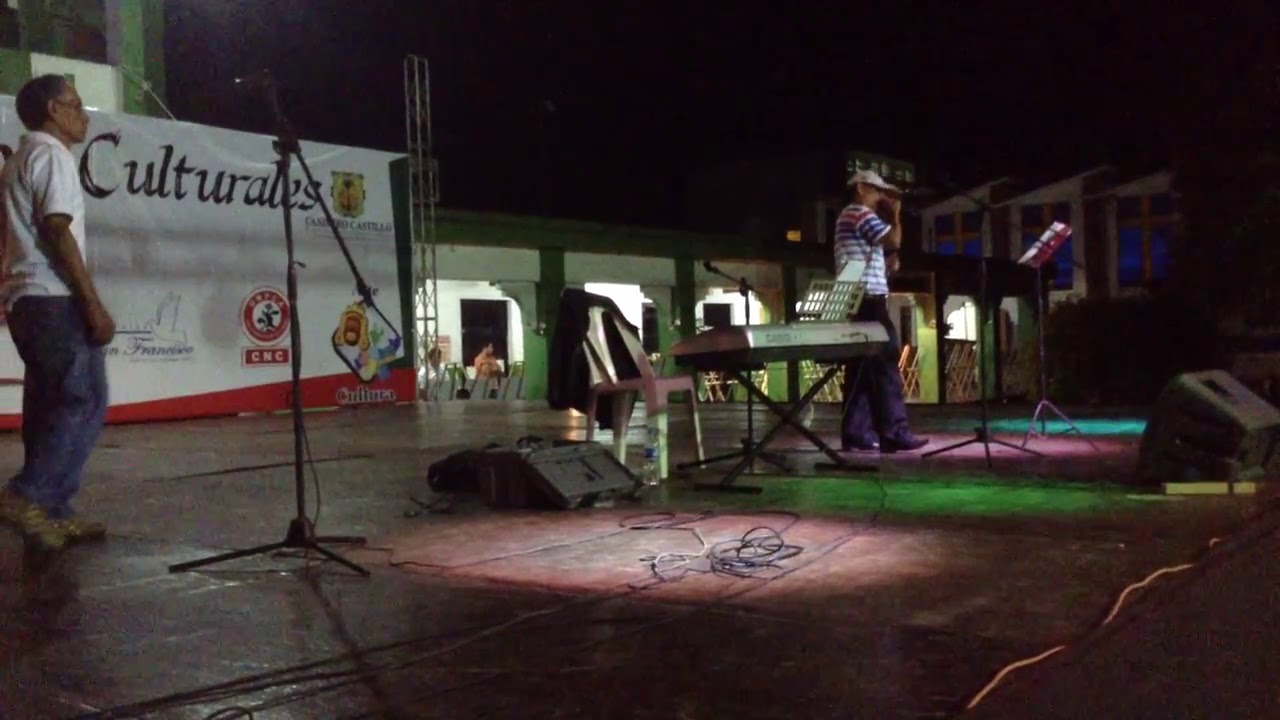The image depicts an outdoor nighttime concert or cultural event. Center stage features a Casio keyboard on a black cross stand, accompanied by a plastic chair with a jacket draped over it. The stage is adorned with a variety of lights—white, green, purple, and blue-green—scattered across the floor, adding a vibrant touch to the dark setting. In the right corner, a black box speaker is angled towards the instruments, with numerous cables trailing across the stage.

Two men are present on stage: one in a striped white and blue shirt with a baseball cap, hands raised near his face, seemingly adjusting a microphone on the left side next to the piano. The other man, wearing a white shirt and blue trousers, is captured walking from the left towards the right. The background showcases a large illuminated sign reading "Culturales," along with various icons and company logos. A brightly lit area and nearby buildings hint at the urban setting of this cultural event, possibly indicating a location like the Philippines.